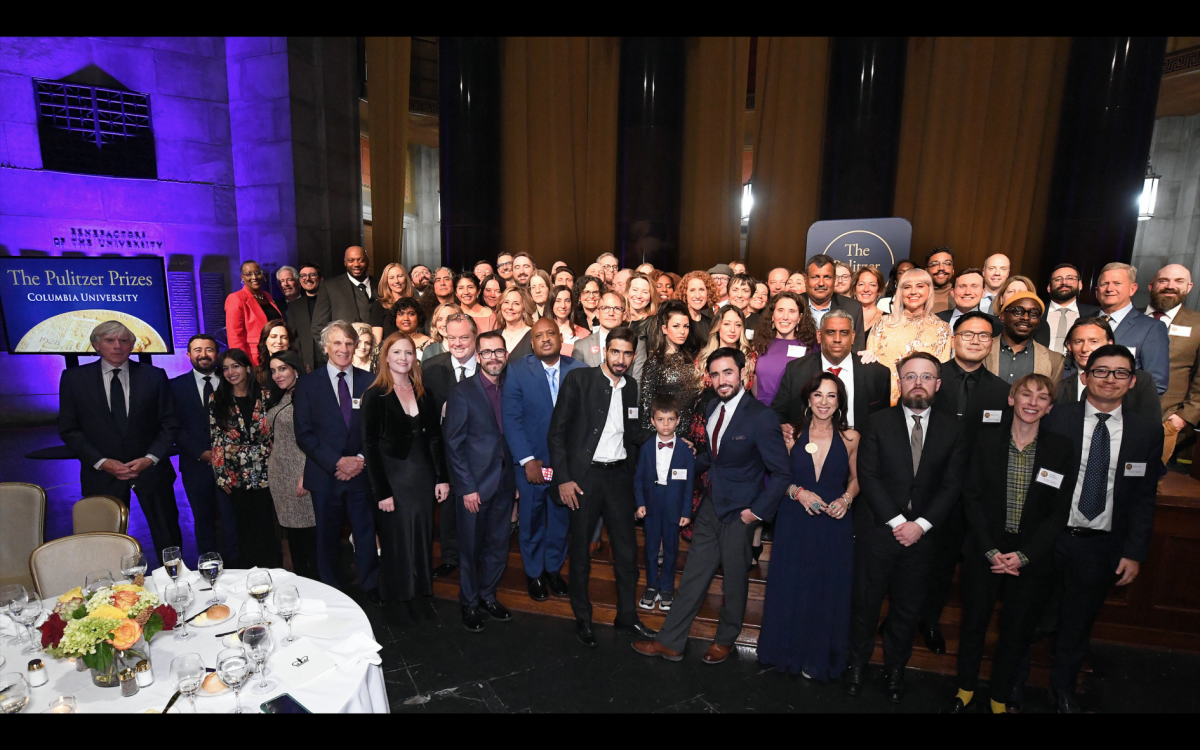This horizontally aligned rectangular photo captures a large group of formally dressed individuals—men in suits and ties, and women in dresses—gathered at what appears to be a prestigious event, possibly a convention or award ceremony. At the center of the image, the group of around 100 people, including adults and one child with a bow tie, are arranged in rows about five to six deep and fifteen across, all wearing name tags. Behind the group, there are large windows adorned with tall theater-like orange-brown curtains, flanked by dark brown wooden panels and interspersed with light fixtures. In the lower left corner of the image, a circular table with a white tablecloth is decorated with glasses, silverware, and a colorful bouquet of flowers. To the left, a purple-lit stone wall features a metal sign indicating "Pulitzer Prizes, Columbia University," suggesting this event is related to the prestigious awards. The scene, embellished with careful decor and dark carpeting, exudes an air of formality and significance.